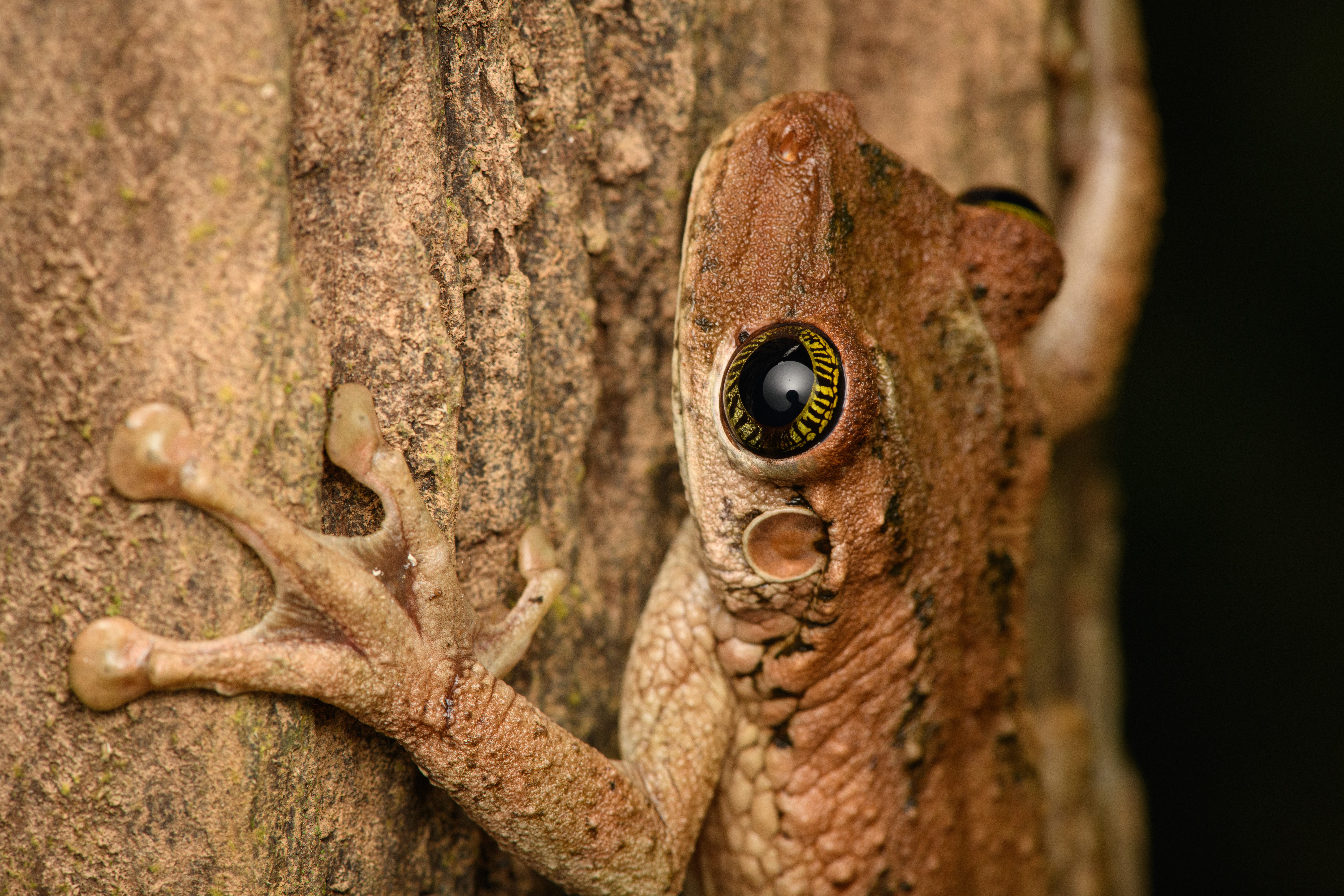This close-up, rectangular photograph, taken in landscape orientation, shows a tree frog closely camouflaged against the textured, brown-and-grey trunk of a tree. The frog's body, featuring a predominantly tan or brown color with faint black spots, blends seamlessly with the sandy tones of the tree bark. Both its arms are prominently visible, with one front leg reaching out and adhering to the tree, showcasing rounded, suction-cup-like toes. The frog's eyes, black with a noticeable yellow-green iris around the edges, stare upwards, reflecting the flash used to capture this nighttime scene. Only the upper half of the frog's body is visible, leaving the hind legs out of the frame. The background is pitch black, highlighting the detailed textures of both the frog and the tree bark.